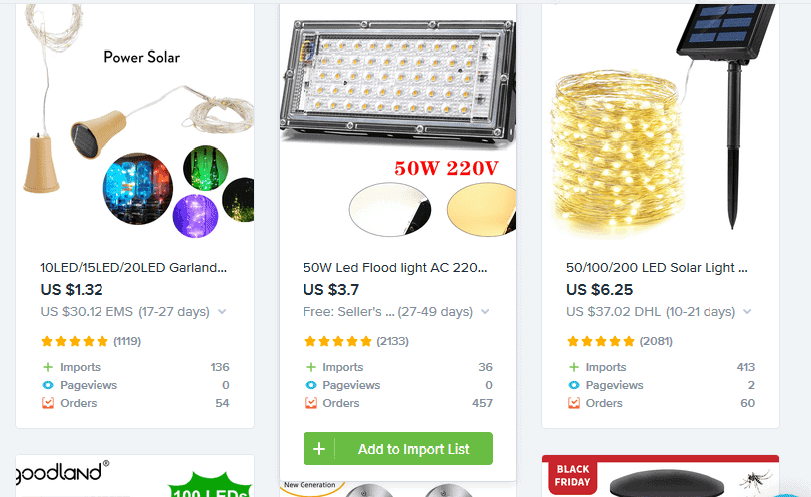**Descriptive Caption:**

The image depicts a detailed screenshot of an e-commerce website showcasing various LED lighting products. The screenshot features three main products: 

1. **Solar-Powered LED Lights**: Offered at an incredibly low price of $1.32. These lights are available in configurations of 10, 15, and 20 LEDs, designed for decorative purposes such as garlands. Despite their affordability, these lights boast a stellar rating with 1,119 reviews and have been imported 136 times with 54 orders placed.

2. **50 Watt LED Floodlight (AC 220V)**: Priced at $3, this powerful lighting solution is designed for broader illumination needs. It enjoys high popularity with an impressive 2,133 reviews, 36 imports, and 157 orders indicating heavy demand.

3. **Solar-Powered Fairy Lights**: These lights, ideal for creating a whimsical ambiance, cost $6.25. They are highly favored, reflected in their 2,081 reviews. The data indicates significant interest with 413 imports and 60 orders. This product is slightly more visible online with two page views recorded.

All three products feature excellent ratings, suggesting strong customer satisfaction. The entries illustrate the high usage and favorable reception of these budget-friendly yet efficient lighting solutions.